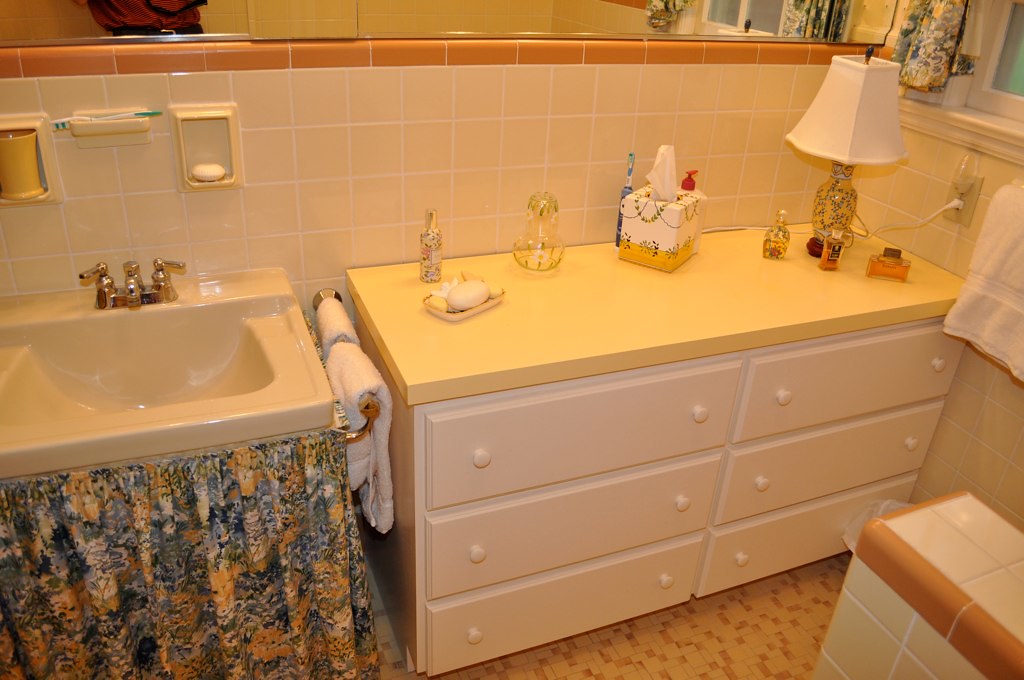This color photograph captures an elegant section of a bathroom artfully decorated with a blend of soft hues and intricate patterns. On the left, a sink graces the frame, its delicate light pink tone complemented by brassy gold fixtures, including a faucet and handles that exude a vintage charm. Hanging neatly in front of the sink is a curtain on a rod, showcasing a beautiful paisley print with accents of orange, blue, and pale pink.

Moving to the right of the sink, a hook holds a pair of large, fluffy white towels, invitingly plush. Adjacent to this, a counter emerges with a vibrant yellow countertop, strikingly contrasting with the adjacent pink tiled wall. Below the countertop are six light pink drawers, adding a touch of cohesive color to the storage area.

At the far right corner of the frame, a stylish lamp with a white lampshade and a gold intricately designed base provides a touch of warmth and illumination. The countertop also features a neatly placed square box of Kleenex, encased in a holder that seamlessly matches the overall color scheme of the space. 

The floor, visible towards the bottom of the image, is tiled in a mosaic of light brown, yellow, and dusty pink tones, rounding off the bathroom's cohesive and aesthetically pleasing decor.